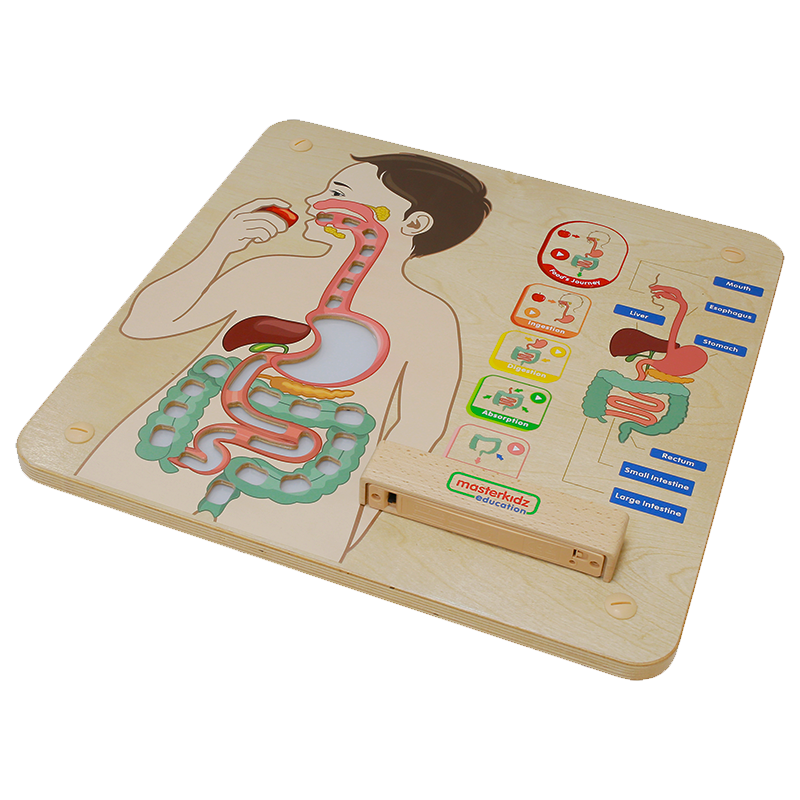The image depicts a wooden educational game board designed to teach children about the human digestive system. At the center of the board, a drawing of a boy with brown hair is depicted starting to eat a piece of red fruit, with a detailed cutaway view showing his esophagus, stomach, liver, and both small and large intestines, outlined in various colors including pink and peach. The light blonde board features the text "Master Kids Education" and contains a right-hand section with informative descriptions about indigestion and the functions of each digestive organ. This section includes labels in blue boxes with white text, identifying the boy's mouth, esophagus, trachea, stomach, liver, rectum, and intestines. Additionally, there appears to be a small remote control-like device on the board, potentially used to highlight different sections of the digestive system for interactive learning.